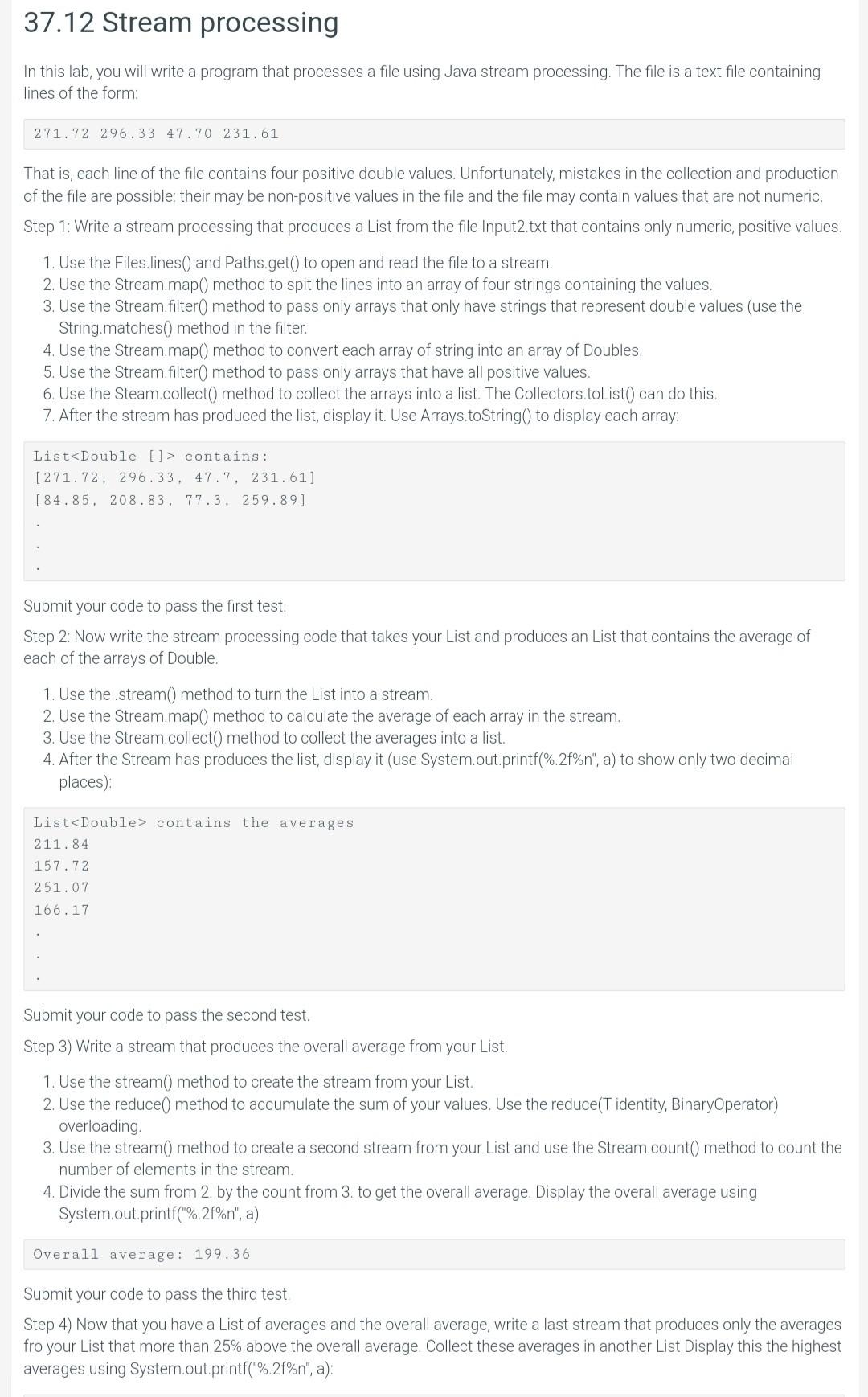The image depicts a printout on a white background, featuring detailed text related to Java Stream Processing. At the top, the heading "37.12 Stream Processing" appears clearly. Below this heading, the instructions guide the reader to write a program in Java that processes a given text file. This text file consists of lines, each containing four positive double values, such as:

```
271.72, 296.33, 47.70, 231.61
```

However, it also mentions potential errors in the file, including non-positive values and non-numeric entries. The first step instructs the user to write a stream processing function that filters out these invalid entries, producing a list of only the valid positive numeric values.

Next, there is a shadowed box filled with numbers, which seems to be more instructions or examples. The next directive is to submit the code to pass the initial test. Following this, the second step asks the user to extend their stream processing code to calculate and produce a list of averages for each array of double values. The page contains seven more steps and an overall tone that suggests it is part of a detailed programming assignment or test.